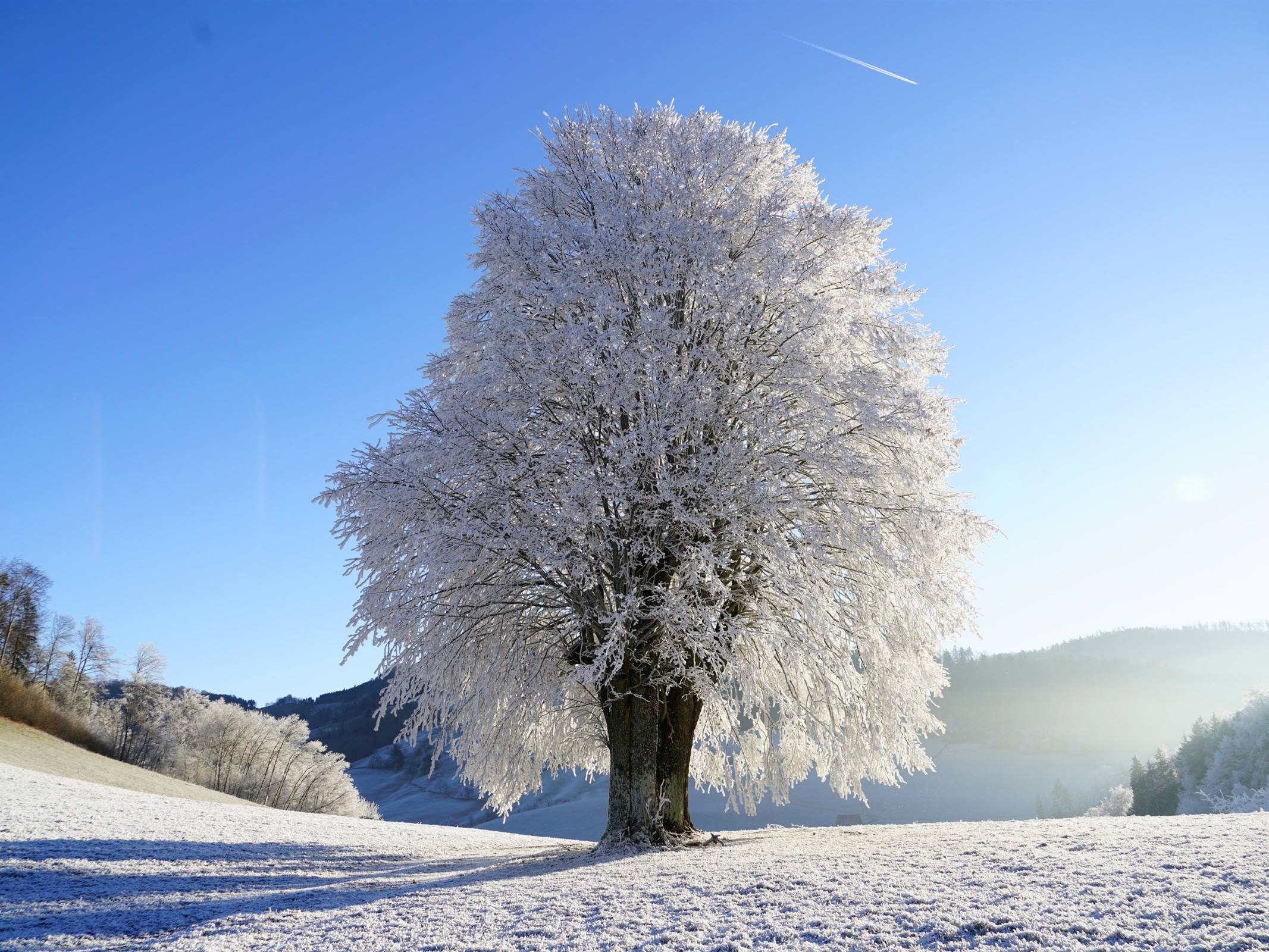In this winter photograph, a magnificent tree takes center stage, its branches coated in heavy ice, giving the illusion of leaves made of ice rather than their usual foliage. The dark trunk and sturdy branches splay out in all directions, weighed down by the frost. The sky behind the tree is a brilliant cornflower blue, accentuated by a white contrail from a passing plane. At the bottom of the image, the ground is blanketed with snow, with bushes to the left similarly iced over and a representation of a forest on the right that extends up a mountain. The scene is illuminated by sunlight, casting a noticeable shadow of the tree on the snow-covered ground, indicating the sun's presence from the top right. The overall effect is a breathtaking winter wonderland, beautifully captured with a clear emphasis on the icy splendor of the scene.